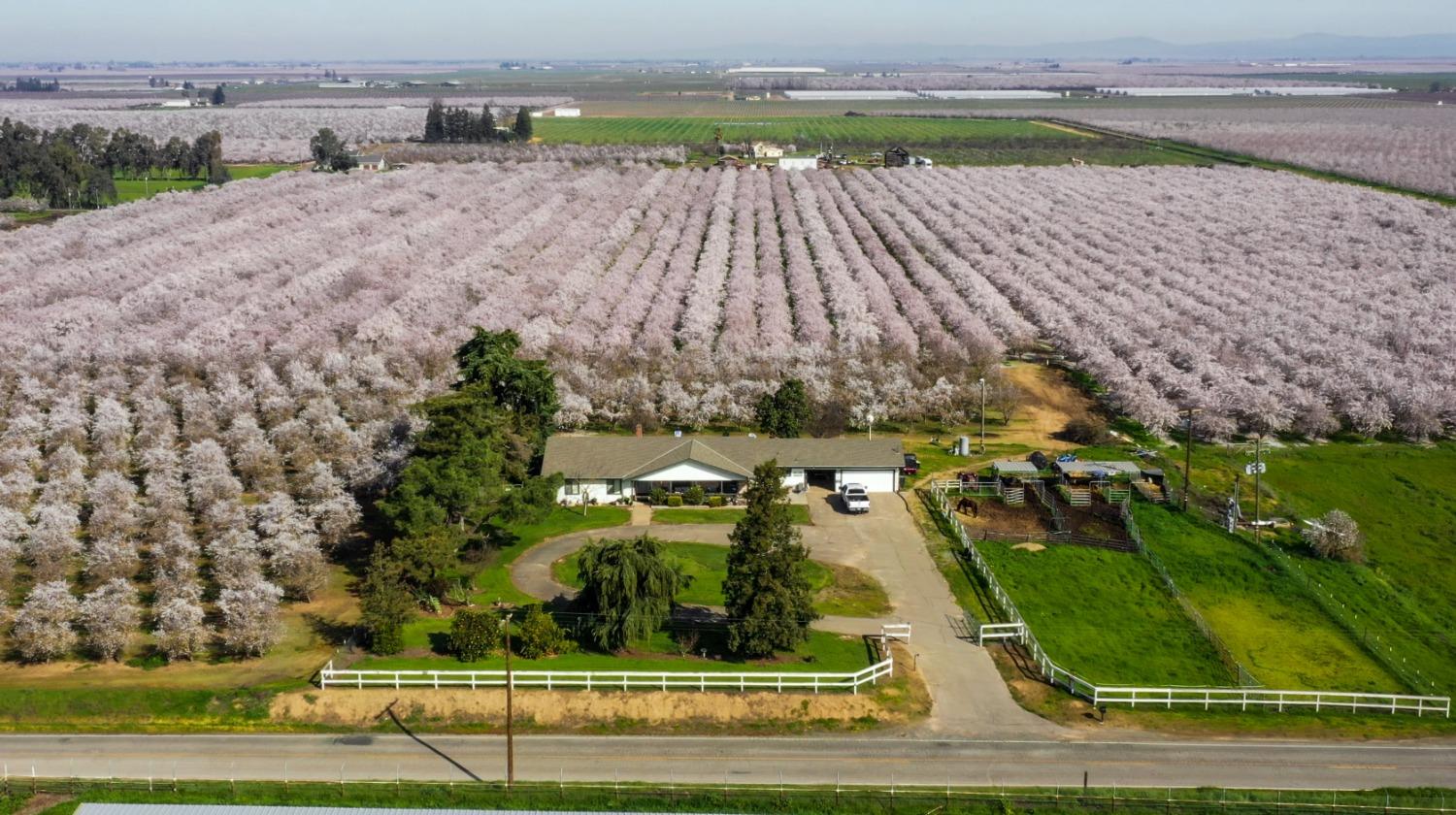This horizontally-oriented, drone-eye view captures a comprehensive scene of a rural landscape. At the forefront, centrally located, is a small, white, one-story farmhouse with a light brown roof. The property features a circular driveway to the left, connecting seamlessly to a regular driveway on the right, where a car is faintly visible. The house is bordered by a white fence, which continues to enclose a green pasture on the right side, occasionally dotted with horses. A picturesque bank of trees lines the left side of the house, creating a natural boundary.

Adjacent to the house in the background are rows upon rows of trees or shrubbery, possibly lilac or cherry bushes, exhibiting a captivating light purplish-pink hue. These tightly packed, flowering rows extend horizontally across the landscape, forming a vivid agricultural mosaic. Further in the distance, additional fields and a grayish, hazy sky define the horizon, adding a tranquil, atmospheric touch. 

The bottom edge of the image is marked by a roadway, along with visible power lines, integrating a touch of modern infrastructure into this idyllic rural setting.